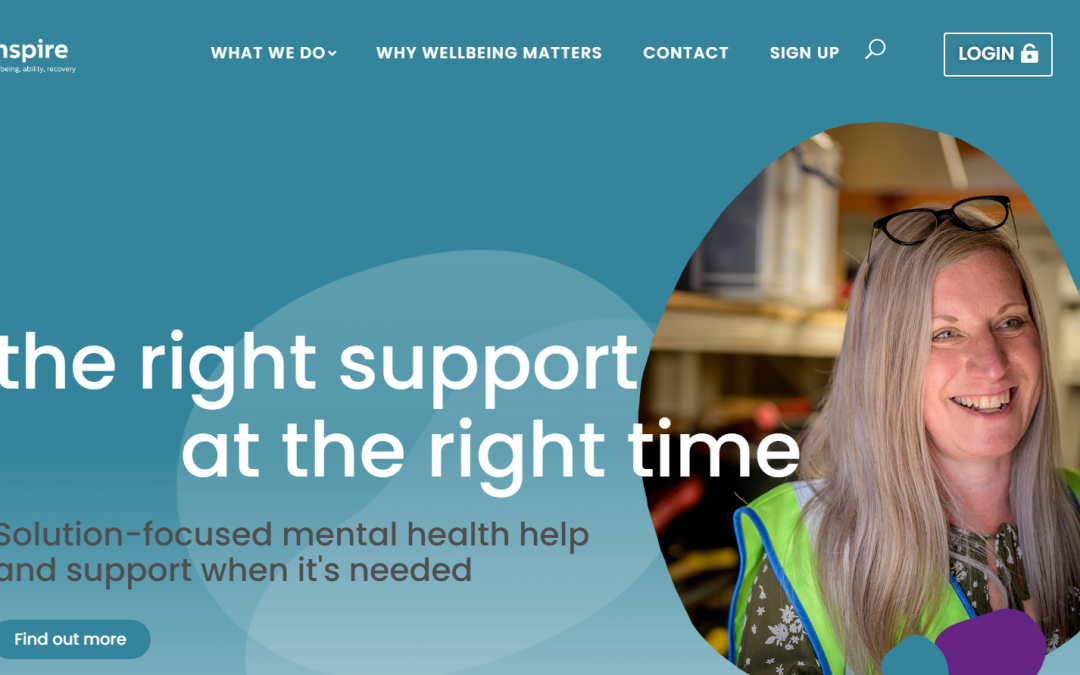The image is a close-up screenshot of a website’s homepage, likely containing the word "Inspire" in its title. The image is zoomed in, making the full website name indiscernible. The top-right corner of the site features several navigation tabs: "What We Do," "Why Well-Being Matters," "Contact," and a "Sign Up" option. Adjacent to these tabs is a search icon, and a login button symbolized by a small padlock. Below these elements is a prominent picture of a woman with silver-gray hair, anchoring the visual focus of the page.